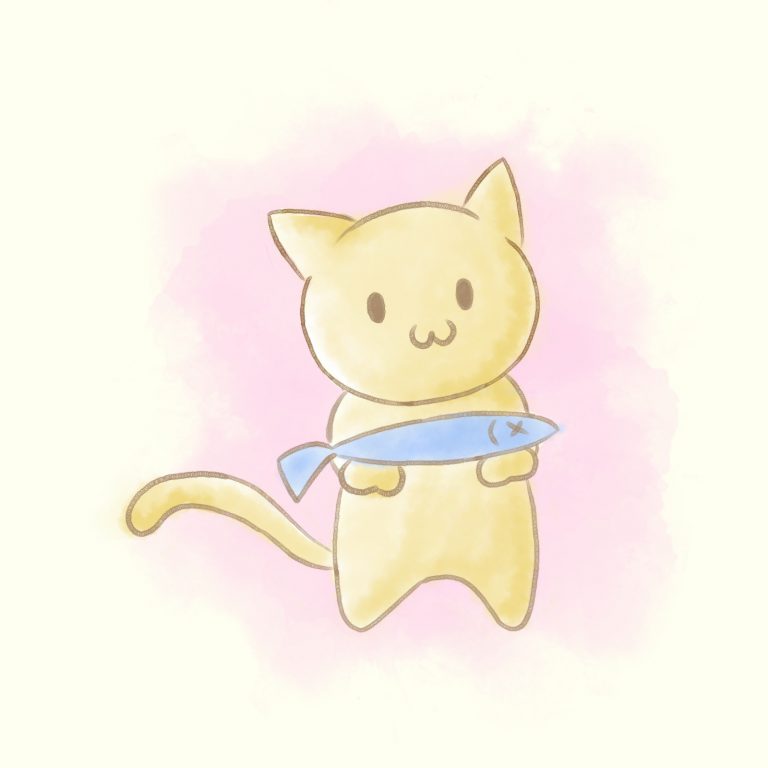In the center of the image is a crudely drawn cat with a round face and pointy ears, combining tan and beige colors. Its facial features are simple: tan dots for eyes and a 3-shaped mouth turned sideways. The cat stands on two legs, holding a blue fish with its paws extended forward. The fish, depicted with minimal detail, has a half-C shape and an X to indicate it is dead. The cat seems joyful, its tail extending to the left from behind. Surrounding the cat is a soft, cloud-like background transitioning from pink to tan, giving the entire illustration a whimsical, cartoonish feel.